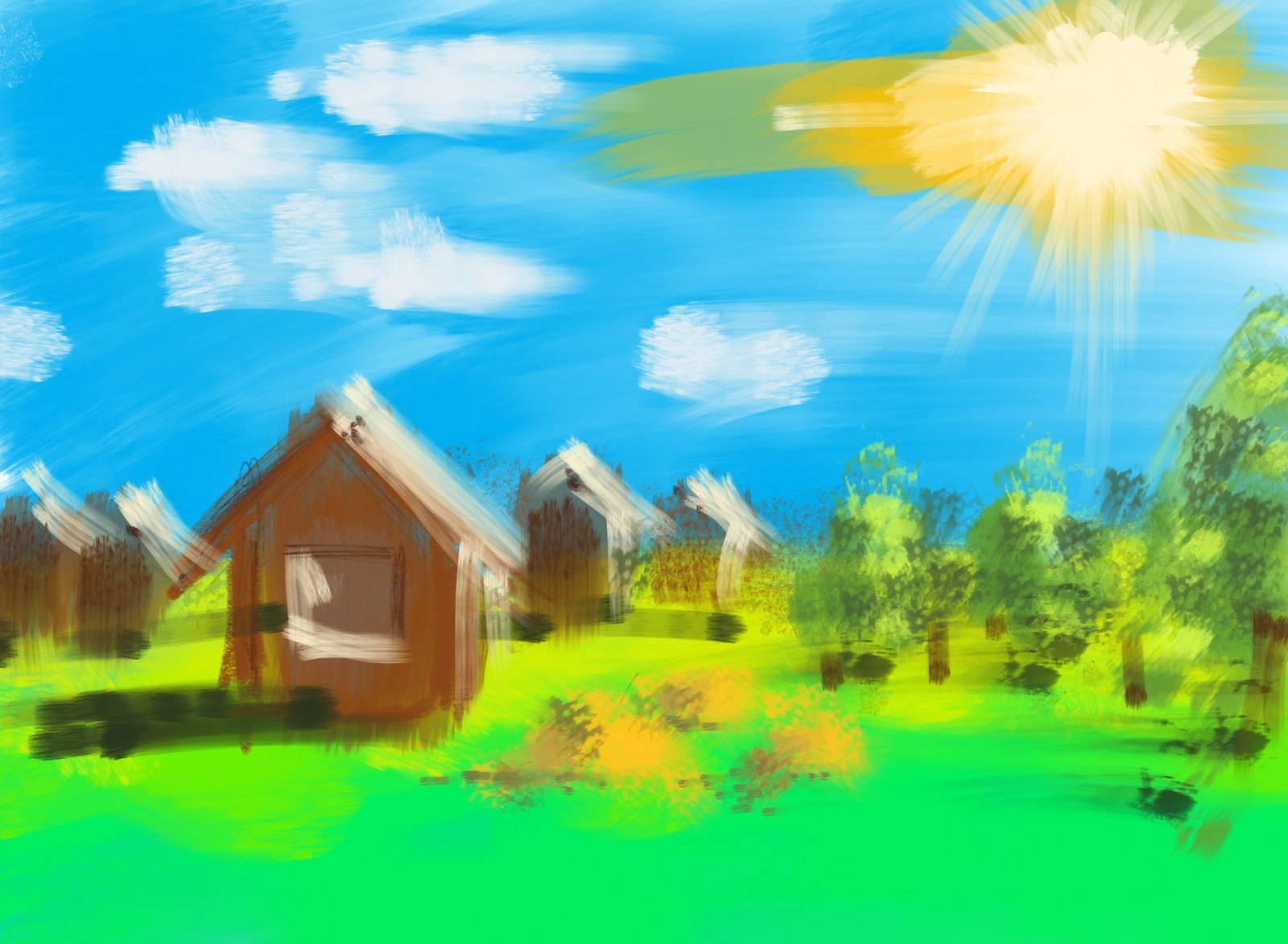This vibrant digital artwork, rendered in a landscape orientation, radiates cheerful energy with its bright and lively color palette. The sky, painted in a vivid blue, is adorned with soft, abstract clouds - a cluster drifting in the top left and a radiant, inviting sun glowing in the top right corner. The scene, though somewhat impressionistic and abstract in style, captures the uninhibited beauty of a sunny day. Dominating the bottom third of the image is a striking field of neon green and neon yellow grass, which pulsates with life and color. To the left, a row of five simplistic, brown houses stand neatly, each with a boxy design, complete with a window and a triangular roof. On the right side, several trees with lush green canopies and sturdy brown trunks add to the idyllic nature of this whimsical landscape.